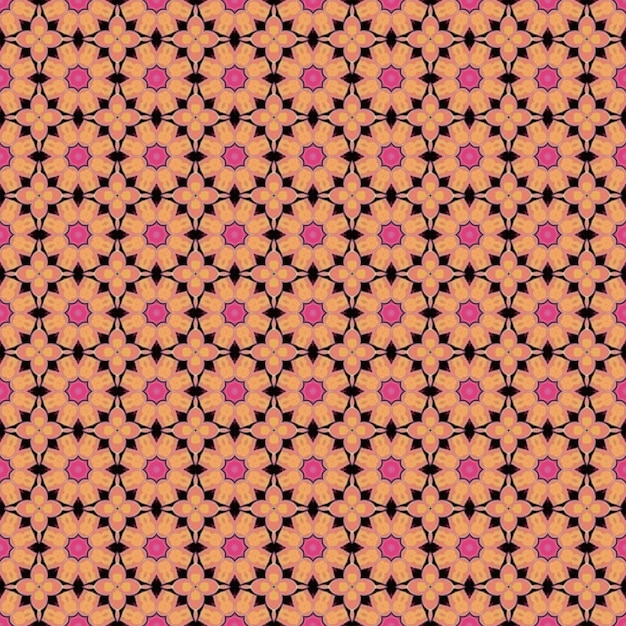This image showcases a highly detailed and repetitive abstract pattern, resembling a stylized floral motif, reminiscent of vintage wallpaper. The central feature of the design is a series of interconnected circles arranged in rows, dominated by a warm orange hue. Each circle houses a hot pink center which contains an even smaller white dot. 

Radiating out from the pink core, the circles are bordered by a darker color, potentially black or an extremely dark blue. Around the edges of each circle are around nine evenly spaced black diamonds that appear to link the circles together in a seamless pattern, giving the impression of an interlocking network. These black diamonds also form double triangles creating a four-leaf design where the circles intersect, adding more complexity to the design.

Between these main circles, smaller, flower-like shapes created from black spaces emerge, each featuring a mix of orange and a moth-like color, positioned diagonally. These secondary patterns add layers to the already intricate design, making the overall composition appear both orderly and richly decorative, perfect for wallpaper that aligns seamlessly, creating a continuous, mesmerizing rhythm across the surface.